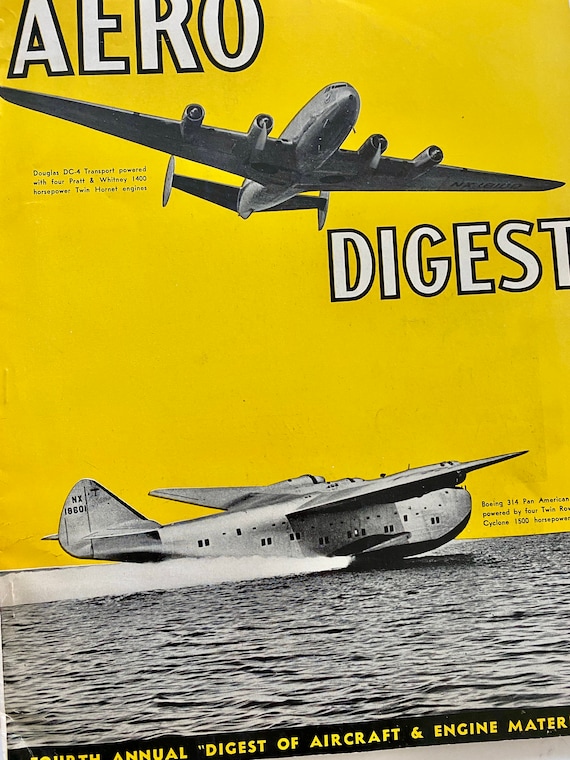The cover of Aero Digest magazine features a vivid, bright yellow background that sets the stage for a striking image of two classic airplanes rendered in black and white. At the top of the cover, the title "Aero Digest" is prominently displayed in white letters outlined in black. Just beneath the title, a large Douglas DC-4 airplane is showcased in flight, emphasizing its front and bottom views. This iconic aircraft is powered by four Pratt & Whitney 1400 horsepower twin Hornet engines. Adding to the intriguing composition, the bottom third of the cover transitions into a black-and-white body of water, where a Boeing 314 Pan American sea plane is depicted having landed. This aircraft is driven by four twin-row Cyclone 1500 horsepower engines and is positioned side-facing, revealing its top and sides. The overall setup is designed to resemble a poster, with additional small text and fine print accompanying the main elements, providing further context on aircraft and engine specifications. The high-quality imagery and detailed descriptions lend an air of sophistication to the magazine's cover.